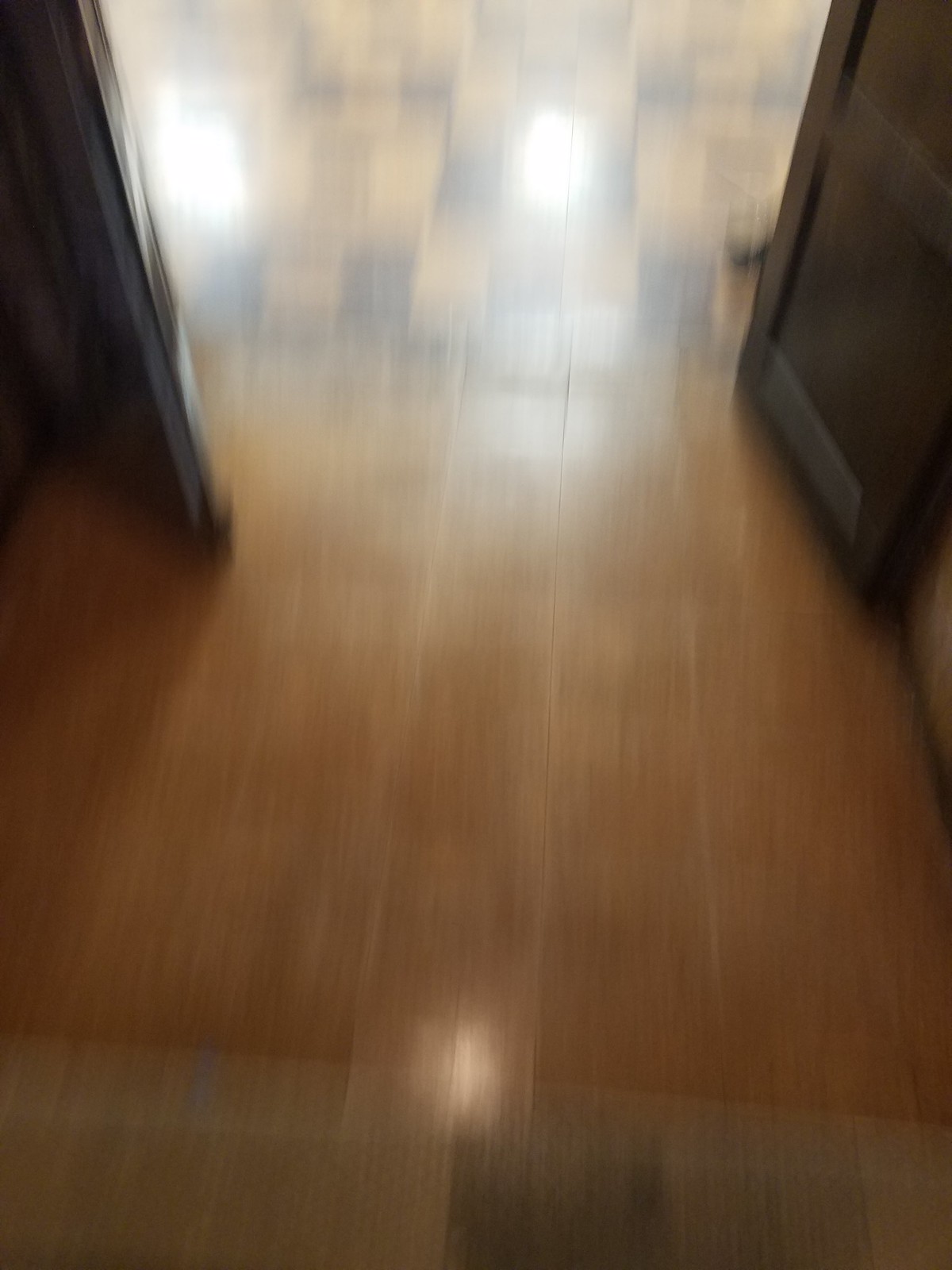This grainy, low-quality photograph captures a section of an interior space, focusing on the floor and an entryway. The glossy, wooden floor in the foreground is illuminated by reflections from ceiling lights, creating a varying sheen across its surface. The entryway features two dark wooden doors, possibly black or deep brown, that open up into an adjacent room. There's no physical threshold between the rooms, but two different floor styles meet at this junction. The room beyond has a checkered tile floor in light blue and white. The poorly defined lines and slight blur make the finer details hard to discern, but the composition and contrasting floor patterns remain apparent. Only the left side of the entryway frame is visible, hinting at another potential door or the frame itself.